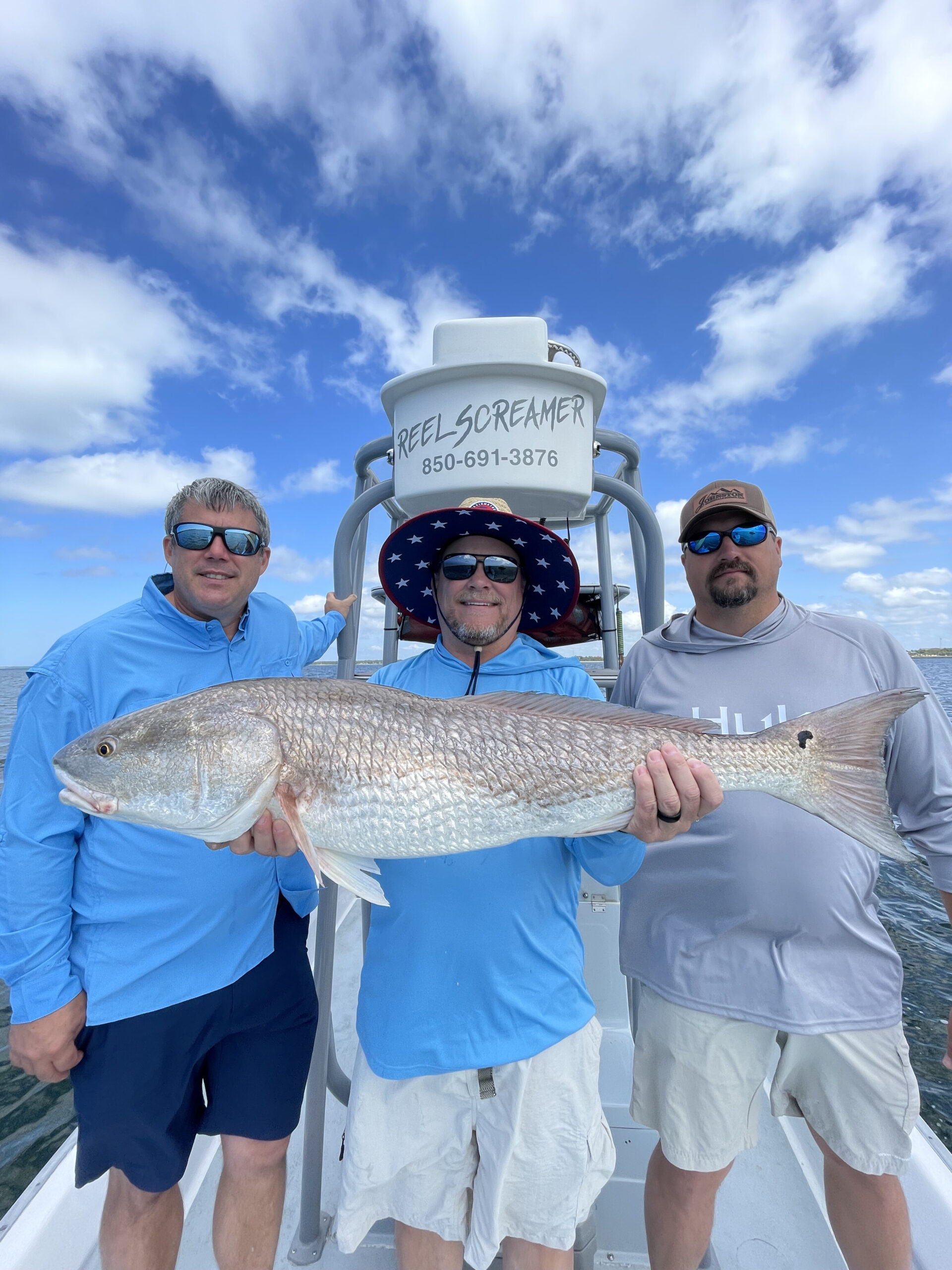The photograph showcases an exhilarating deep-sea fishing experience, possibly an advertisement for a fishing boat lease. Titled "Real Screamer," the name is prominently displayed along with a phone number for chartering this fishing adventure. The image centers around three middle-aged, white men standing side by side on the boat, cropped just below their knees. 

In the middle, a man proudly presents a massive fish that resembles a grouper or a spot fin. He wears a light blue long-sleeve shirt, white shorts, a distinctive hat with an inner brim patterned with dark blue and white stars, and reflective sunglasses. Flanking him on the left is another man in a light blue long-sleeve shirt and dark blue shorts, wearing reflective sunglasses and a baseball cap, along with a gray hoodie-style shirt. On the right stands the third man, sporting a gray long-sleeve shirt, white shorts, and reflective sunglasses.

The backdrop features a clear, blue sky adorned with wispy clouds, indicating a windy day on the water. Together, these elements create an enticing visual for deep-sea fishing with Real Screamer, perfectly capturing the excitement and rewards of the experience.